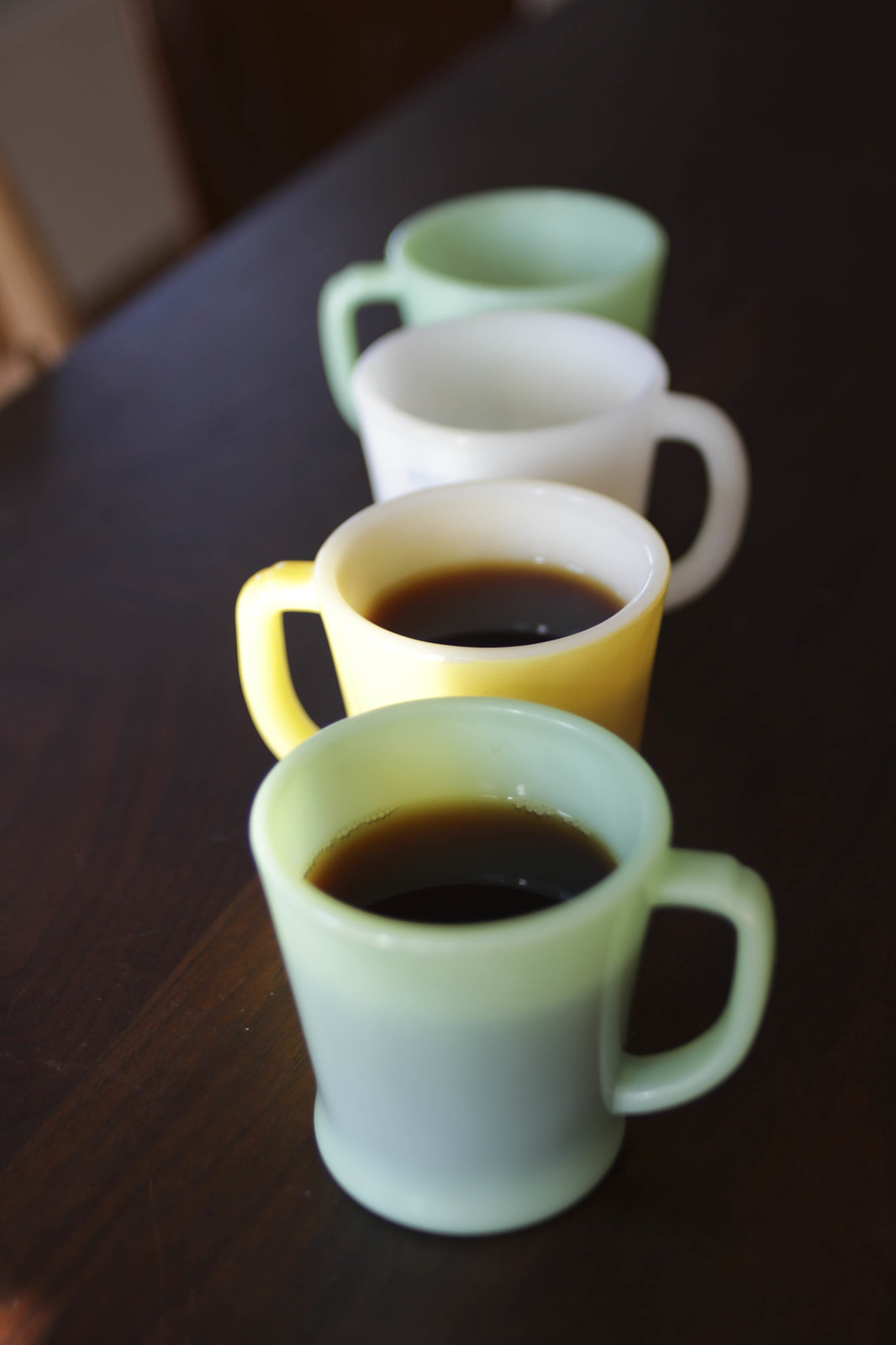The photograph features four coffee cups arranged vertically in a straight line from the viewer's perspective, diminishing towards the top of the image. The cups sit on a dark brown wooden table. The first cup, closest to the viewer, has a light green tint and is nearly full with a brown liquid, slightly translucent to reveal some details. The second cup is yellow with a white interior, showing a slight translucence on one side with visible coffee inside. The third cup is pure white with no visible liquid, and the fourth cup is a pale green, also without visible liquid. The cups' handles alternate sides: the first to the right, the second to the left, the third to the right, and the fourth to the left. The background includes an out-of-focus white wall with brown trim and a brown door, mostly cut off from the frame. The overall focus of the image sharpens on the closest cups and blurs progressively towards the background.